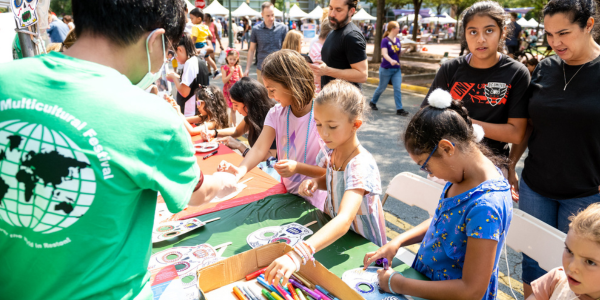This photograph captures a vibrant street fair or outdoor school event, likely a craft fair or festival, bustling with activity. The central focus is on a group of children, mostly girls aged around six to nine, seated at a long table engrossed in various crafting activities. They are coloring paper skulls mounted on popsicle sticks using an assortment of crayons and markers from a cardboard box, with one girl prominently reaching for a marker. A boy in a green shirt and face mask stands nearby, observing the table. Behind them, the scene is set against the backdrop of numerous white tents arranged in a row under a bright, sunny sky. Several adults, including one woman in a green t-shirt with a globe design, are present, either supervising the children or mingling in the background. The lively atmosphere is complemented by the presence of other tables and clusters of people, suggesting a larger community gathering or school event. In the upper right corner of the image, a young lady stands beside a woman who could be her mother, both captured glancing towards the camera, adding a personal touch to the communal scene.